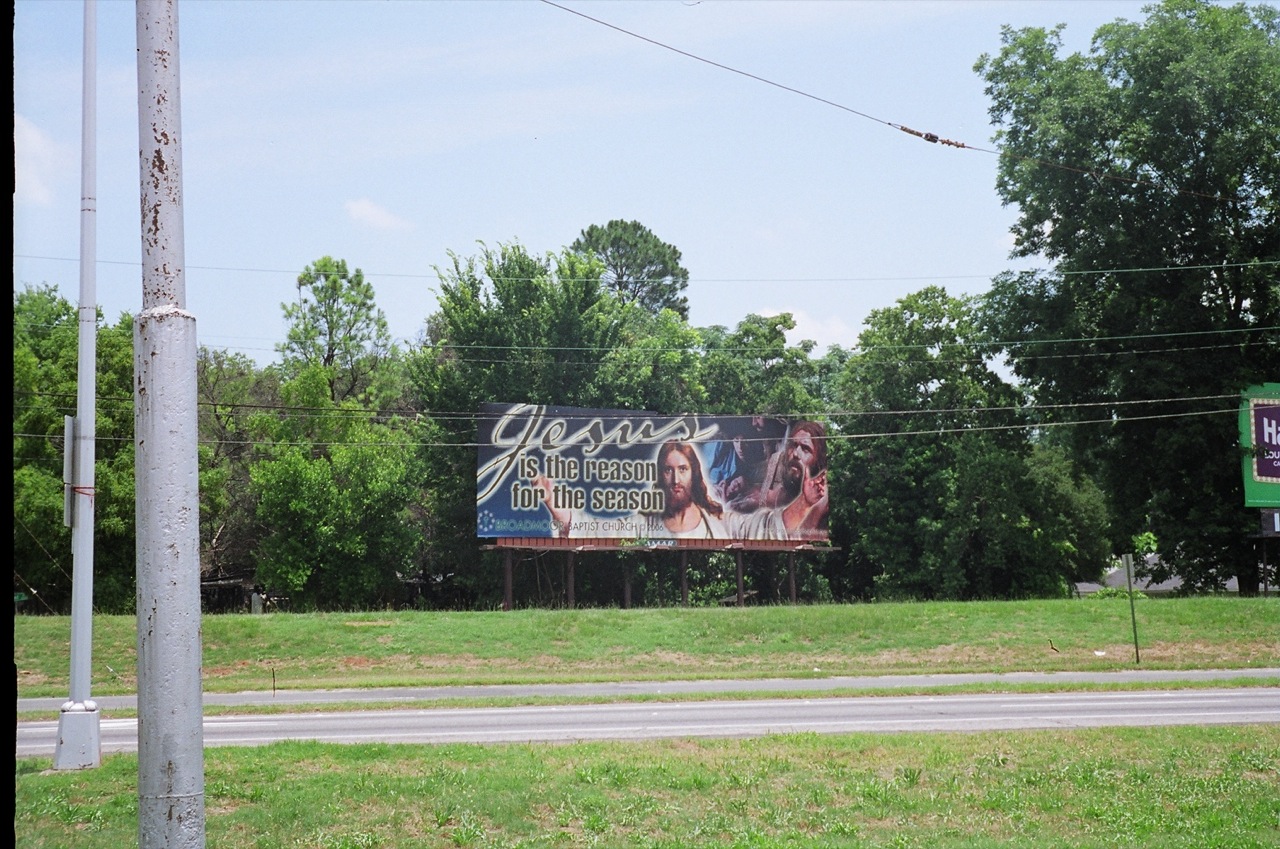The photograph captures an outdoor scene with an overcast blue sky scattered with white splotches. Dominating the background is a dense line of dark green trees. In the foreground, a gray road, divided by a grassy median, leads in opposite directions. On either side of the road, the grass is light green with patches of gold and brown. The scene is further detailed with two large silver poles and small white utility lines.

To the left stands a prominent billboard, mounted on metal poles with a rusty appearance. The billboard, on a dark blue background, reads in cursive, "Jesus is the reason for the season," and features an image of a light-skinned Jesus with long brown hair and a beard, dressed in a white robe with his arms outstretched. A close-up of Jesus and other figures can be seen to the right. The billboard's text is highlighted with a white edge, making it stand out against the blue backdrop. Additionally, a smaller section of the same billboard edge appears on the right side of the image, along with more dark green trees, completing the serene yet pensive scene.